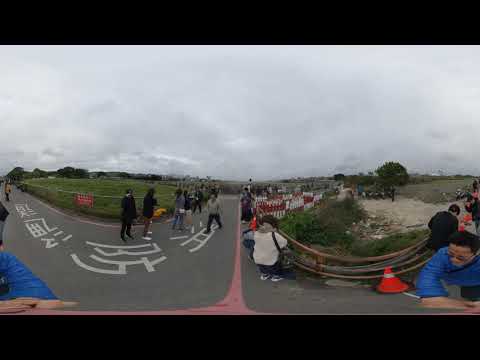In this detailed image, a scene from an outdoor setting in an Asian country is depicted on a cloudy day. The image is framed by solid black borders at the top and bottom. Below the top black border, the sky is densely filled with clouds. At the bottom, a narrow road or walkway, possibly a racetrack, runs through the image with an Asian language written on it. This pathway curves in two directions and is the central feature, drawing a crowd of people walking along it. 

On either side of this path, there are metal fences and railings, with a red sign visible on the railing to the right. The left side shows someone painting lines or possibly words on the pavement, while others stand around conversing. This road is bordered by a stripe, and there's a curved fence on the right to prevent people or vehicles from cutting across the adjacent sand strip.

Lush green patches of grass, trees, and bushes are scattered throughout. The image captures vibrant colors including black, white, gray, green, red, blue, yellow, orange, maroon, and a hint of purple.